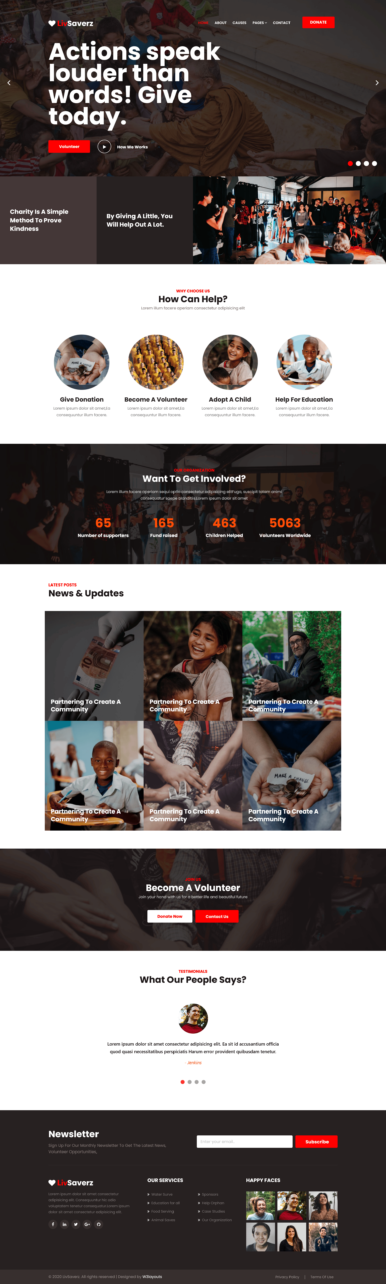The image depicts a series of screenshots from a website with a distinctive layout and various sections. At the top, the screenshot features a black background with "Live Savers" prominently displayed in the upper left-hand corner. Below this, several menu headers are visible. Centrally, in large white text, the motto "Actions Speak Louder Than Words! Give Today" is highlighted, followed by a prominent red donation button. 

Beneath this section, there are four boxes arranged horizontally. The first box, on the left, is light gray with white text, while the second box to its right is dark gray with white text. The third box appears to feature an image of several people gathered around a couch, most of whom are dressed in black shirts. The fourth box is not described in detail.

Below these boxes, a white box contains four circles arranged in a row, centered by the text "How Can Help?". Each circle contains a different image: the first shows a hand holding a book, the second depicts a field of crops, the third features a young girl in a short-sleeved shirt, and the fourth shows a student in a short-sleeved white shirt.

Following this, a black box with the text "Want to Get Involved?" is shown, alongside four numerical columns. Beneath this box are six pictures arranged in two rows and three columns, presumably related to the organization. 

Another black box, beneath these images, reads "Become a Volunteer" and contains both a white button and a red button. Moving further down, a white box with the heading "What Are People Say?" features a circle with a person and a quote attributed to them.

At the bottom of the screenshot, a black box includes a newsletter sign-up and a search bar. In the lower right corner, six additional images are arranged in two rows and three columns. The term "Live Savers" is repeated in the bottom left corner of this section.